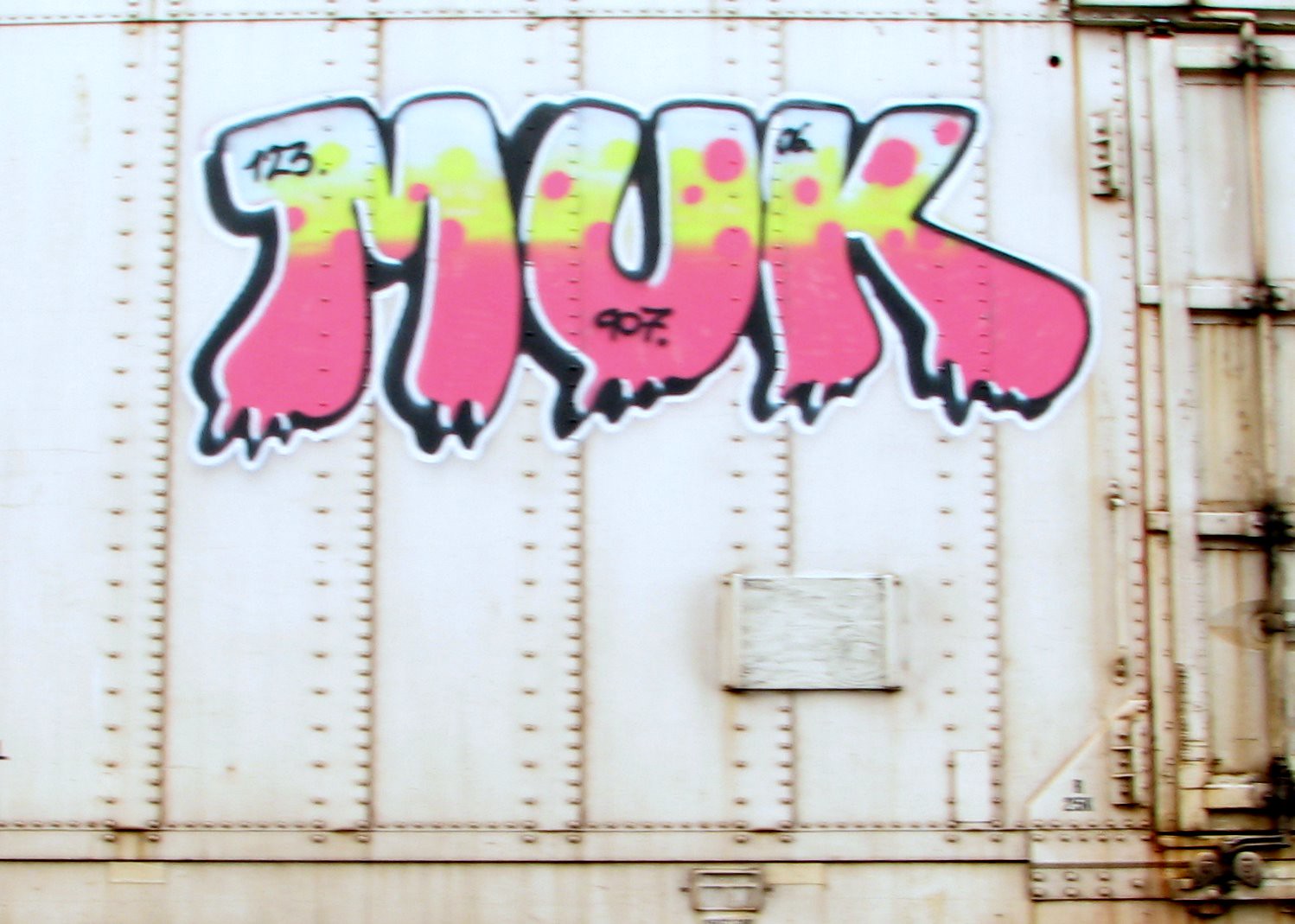This image captures a close-up view of the side of an old, white metal train car, showcasing intricate graffiti art. The train car, which appears aged and weathered with rivets and a yellowish-brown tint resembling rust, features prominently in the shot. Central to the image is a large, colorful piece of graffiti spelling out "MUK" with dynamic 3D black and white lettering. The letters of "MUK" are accentuated with vibrant touches of pink at the bottom and yellow in the middle, creating a striking visual effect with pink dots extending into the whitish area of the 'M'. The graffiti includes smaller elements, with the numbers "123" visible under the 'U' and "90706" incorporated within the design. The overall scene is rich with texture and color, highlighting the artistic embellishments on the aged, industrial canvas of the train car.